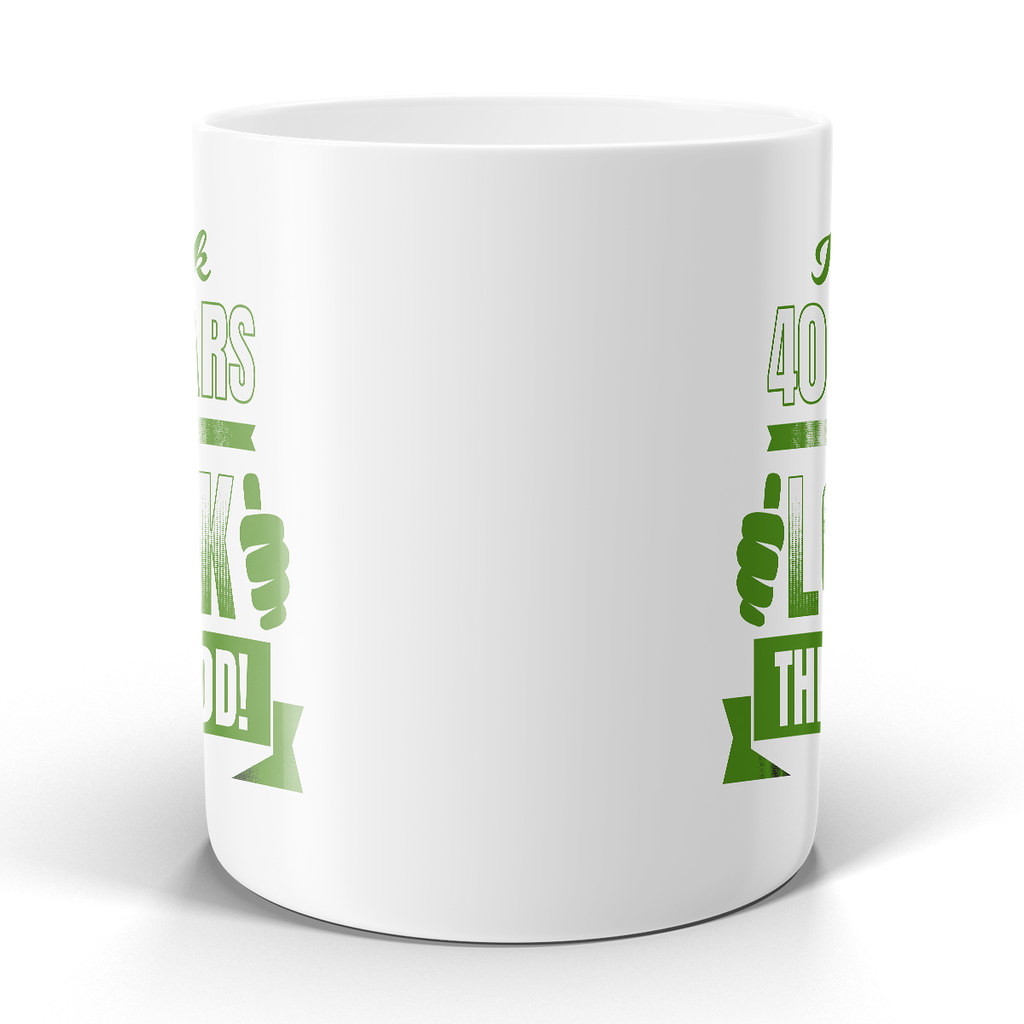This close-up photograph features a white ceramic coffee mug set against an entirely white background and surface, creating a bright and well-lit image. The mug casts a subtle shadow beneath itself, adding depth to the composition. The handle of the mug is not visible, likely positioned on the far side away from the camera. The mug features a partially visible green text graphic. On the right side of the mug, the text reads "40" followed by an "L" underneath a green line and a banner with "TH" in white font within it. The left side of the mug shows the letters "RS," "K," "OD," and an exclamation mark. Additionally, there is a green ribbon-like element at the bottom of the mug's design.